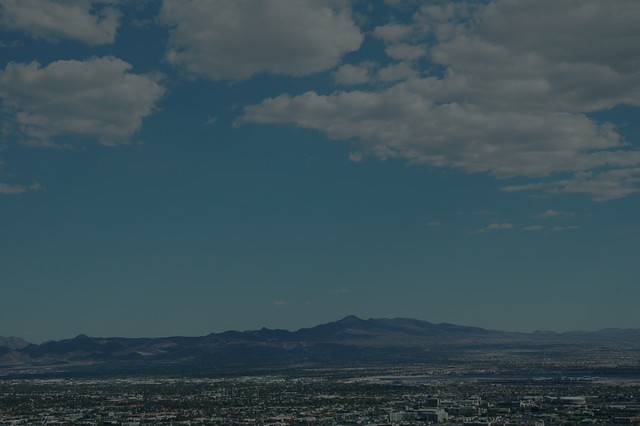This color photograph presents a serene outdoor vista encapsulating both natural and urban elements. The lower fifth of the horizontally-oriented rectangular image showcases a cityscape adorned with low-rise buildings and abundant trees, suggesting a desert community. In the background, a modest mountain or hill, partially covered in foliage, punctuates the horizon. The broad expanse of the scene captures a bright blue sky adorned with white clouds. Despite the apparent sunshine, the overall lighting appears muted and dark, potentially due to the image's quality. High in the sky, the sun's position casts discernible shadows, particularly noticeable in the reflection and shadows of clouds on the right side of the photograph. The harmonious blend of man-made structures and natural beauty creates a captivating and detailed portrayal of this tranquil desert landscape.